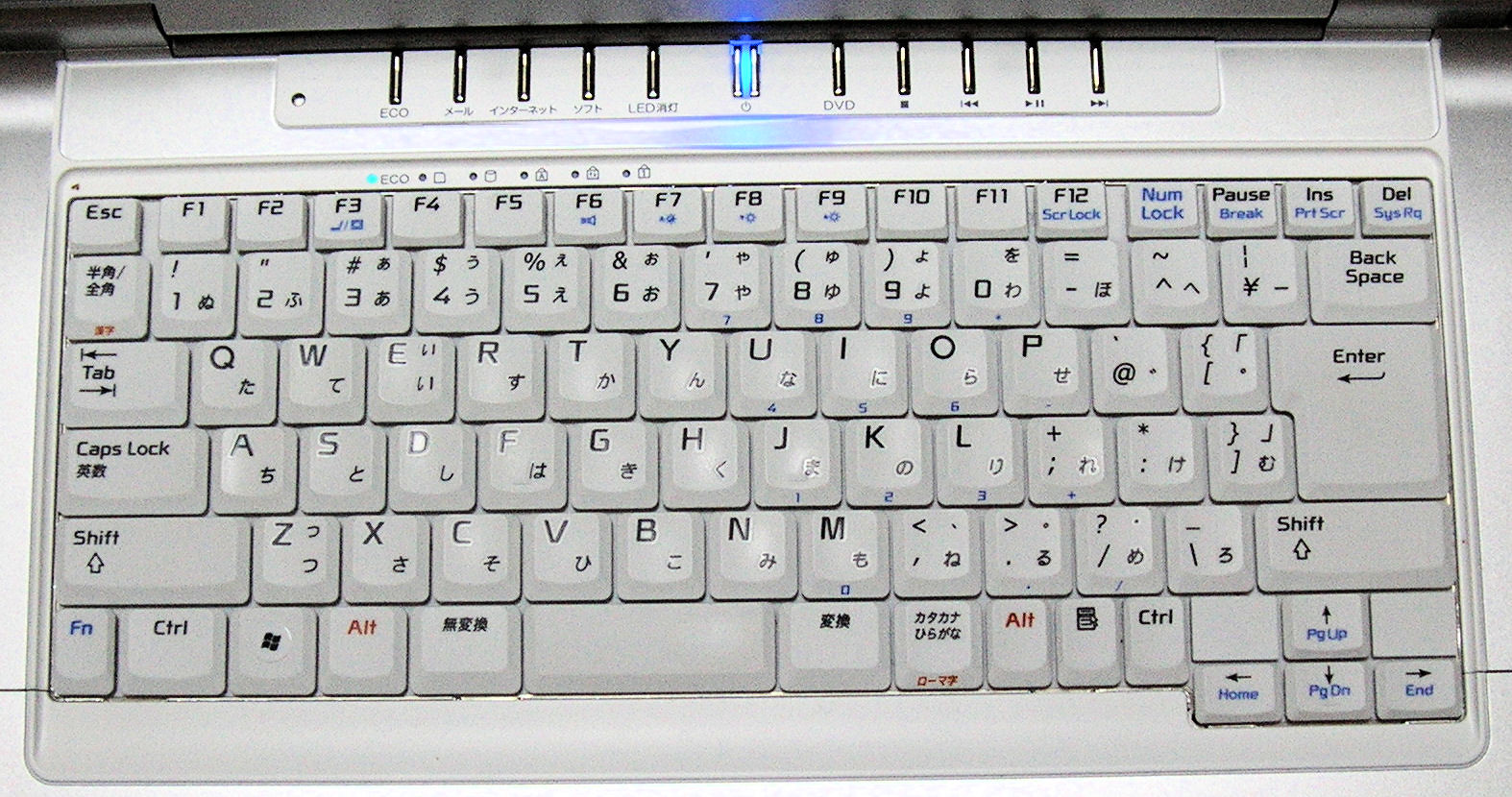The image displays a compact keyboard primarily in white with black lettering, along with scattered accents of dark blue and red, especially noticeable on the ALT buttons. The keys appear slightly raised, and in the top center is a prominent light blue power symbol, emitting a notable blue hue that reflects on the keyboard's surface. Surrounding this blue light are five buttons on each side, each bearing both English labels such as "DVD", "LEFT", "LED", and "ECHO" and others in a different language. Notably, this keyboard lacks a separate numeric keypad, adhering to a more streamlined layout suited for compact use. Additionally, it appears to be part of a possible laptop setup, seated on a silver or gray metallic surface, and equipped with various function keys including ESC, F1-F12, NUM LOCK, PAUSE, INSERT, and DELETE.